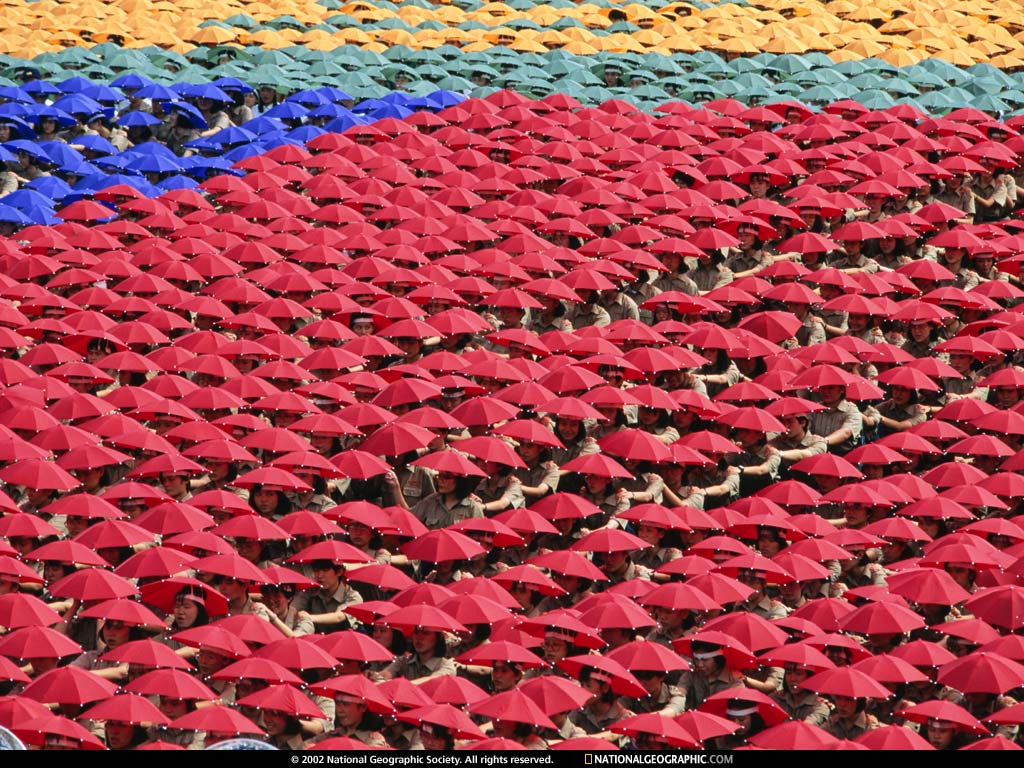This photograph, taken by the National Geographic Society and copyrighted either in 2002 or 2007, depicts a spectacular visual scene composed of hundreds of people standing closely together in line formations. The bottom of the image features a black banner with white text that reads "All Rights Reserved" along with the National Geographic logo and "NationalGeographic.com". 

The crowd predominantly features individuals wearing umbrella hats, presenting a mesmerizing sea of mostly red umbrellas. Among the red umbrellas, there are patches of blue, teal, yellow, and even some purple, creating a vibrant mosaic of colors. The individuals are seen wearing park ranger-like tan, short-sleeved button-up shirts, and some have their hands placed on the shoulders of the person in front of them, suggesting a coordinated effort or possibly a parade formation. The exposed faces indicate that many of the participants are Asian women. This vivid assembly could be intended for an overhead visual display, possibly forming a moving image or part of a collaborative artistic performance.